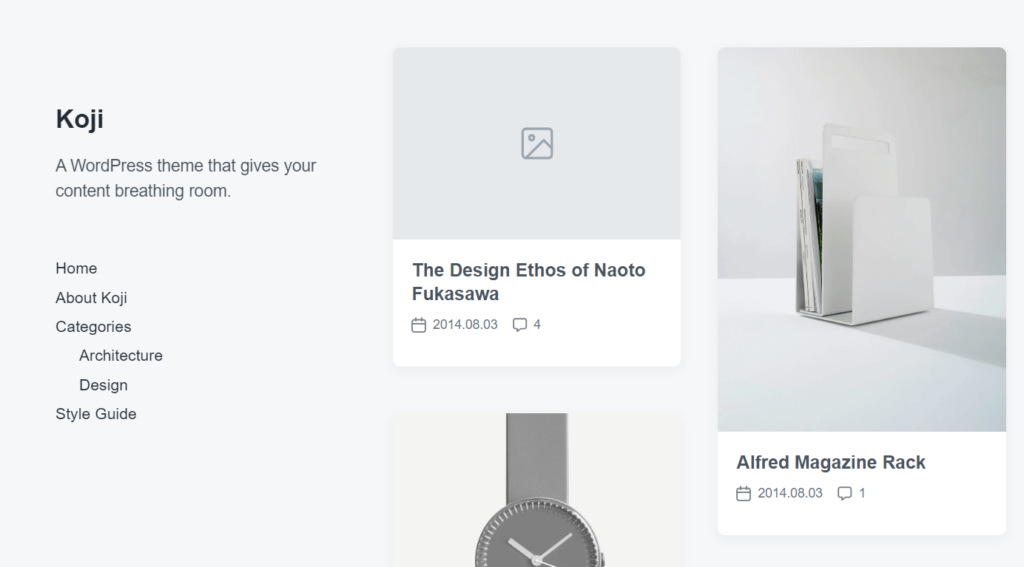This is a cropped screenshot of a WordPress theme named "Koji," featuring a minimalist and clean design. The background is predominantly gray, and at the top left corner, the theme name "Koji" is displayed in bold black letters. Directly beneath it, the tagline "a WordPress theme that gives your content breathing room" is written in small black letters. A vertical category list is present on the left side of the page, featuring links labeled Home, About Koji, Categories, Architecture, Design, and Style Guide.

On the right side of the page, there are three sections showcasing content or products. The top left section contains a blank placeholder image with a gray background and a photo emoji in the center. Below this image, a white box displays the title "The Design Ethos of Naoto Fukasawa" along with a calendar icon and date on the left, and a chat icon with the number four on the right.

Further down the page, a partial view of a black watch is shown on the bottom left. The rest of the watch, including its description and associated icons, is cropped out of the screenshot.

To the right, a large rectangular section features an image of a file folder system. Below the image, a white box with bold black lettering reads "Alfred Magazine Rack." Underneath this box, a calendar icon with the corresponding date is displayed on the bottom left, alongside a chat icon with the number one on the right.